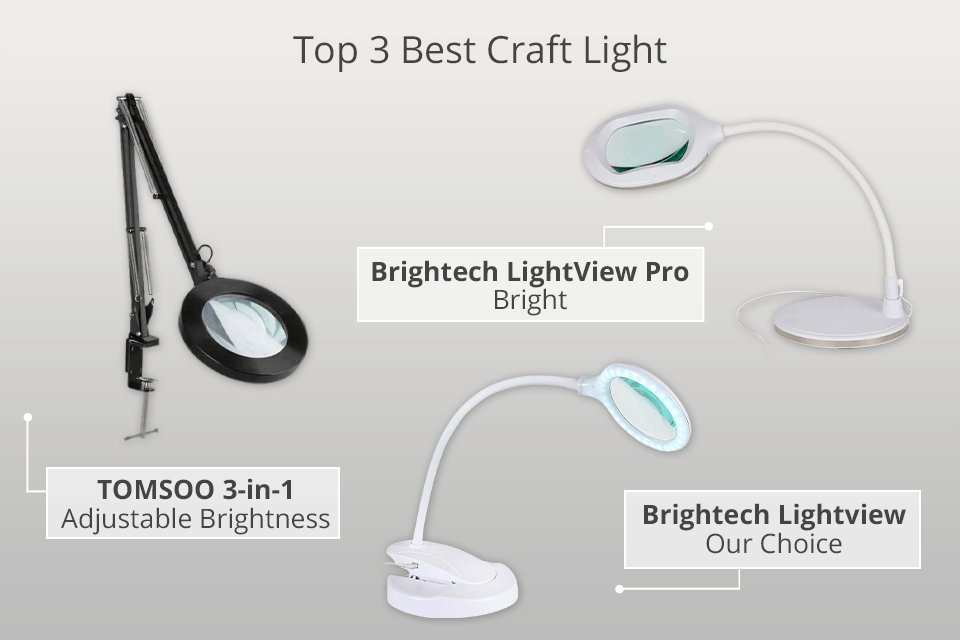**Top Three Best Craft Lights for Precision and Convenience**

This image showcases the top three craft lights ideal for activities requiring high visibility and fine detail work, such as sewing and other arts and crafts projects. 

1. **Brightech LightView Pro**: At the top of the image is the Brightech LightView Pro. It features a small white platform with an extendable, flexible coil, and includes an illuminated mirror. The box beneath the device highlights its "brilliant" lighting capabilities, making it perfect for tasks demanding high brightness.

2. **Tomsoo 3-in-1 Adjustable Brightness**: The second recommended light is the Tomsoo, identified by its unique clamp feature. Unlike the freestanding Brightech, the Tomsoo has a vice-like clamp and a screw-on handle, allowing it to attach securely to table edges or other surfaces. This ensures stability and versatility in placement.

3. **Brightech LightView (Our Choice)**: The final and overall recommended light is the Brightech LightView. This model combines the best of both worlds with a clip mechanism that ensures it can be attached or positioned securely without the need for a vice or just relying on a flat base.

The background features a gradient effect, starting from a light gray at the top and transitioning to a darker gray towards the bottom, adding a clean and professional look to the presentation.

Overall, these lights are praised for their adjustable brightness and convenient design, catering to various crafting needs and environments.